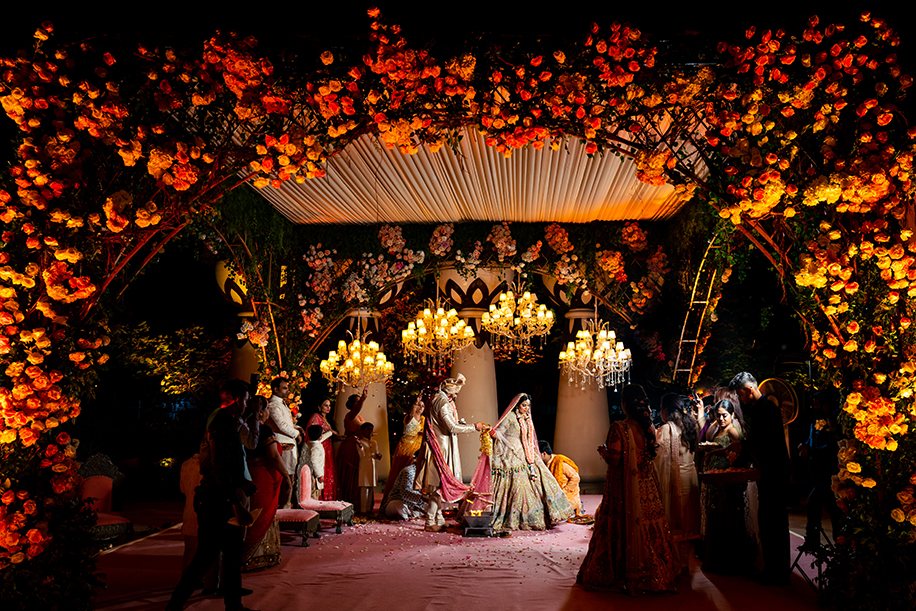In this vibrant photograph of an Indian wedding ceremony, the bride and groom stand in the center of a dark venue, beneath a canopy of flowers and sling lights that bathe the scene in a warm, orange-yellow glow. The ceiling is adorned with a stunning array of flowers, primarily orange and yellow, creating a lush, floral canopy that adds to the festive atmosphere. Below, the floor is covered with rich red fabric, matching the two low, red velvet chairs positioned on the left side of the room. The couple is elegantly draped in a long red fabric, symbolically connecting them.

Suspended above them are four large, illuminated chandeliers that cast a soft light over the scene. Around the couple, a small crowd of people gathers, their figures mostly in shadow save for one woman, whose face is visible with her dark hair parted and slicked back. Despite the dim lighting, the celebratory mood is palpable, enhanced by the presence of autumn-colored floral decorations and the sense of an intimate gathering witnessing a significant moment.